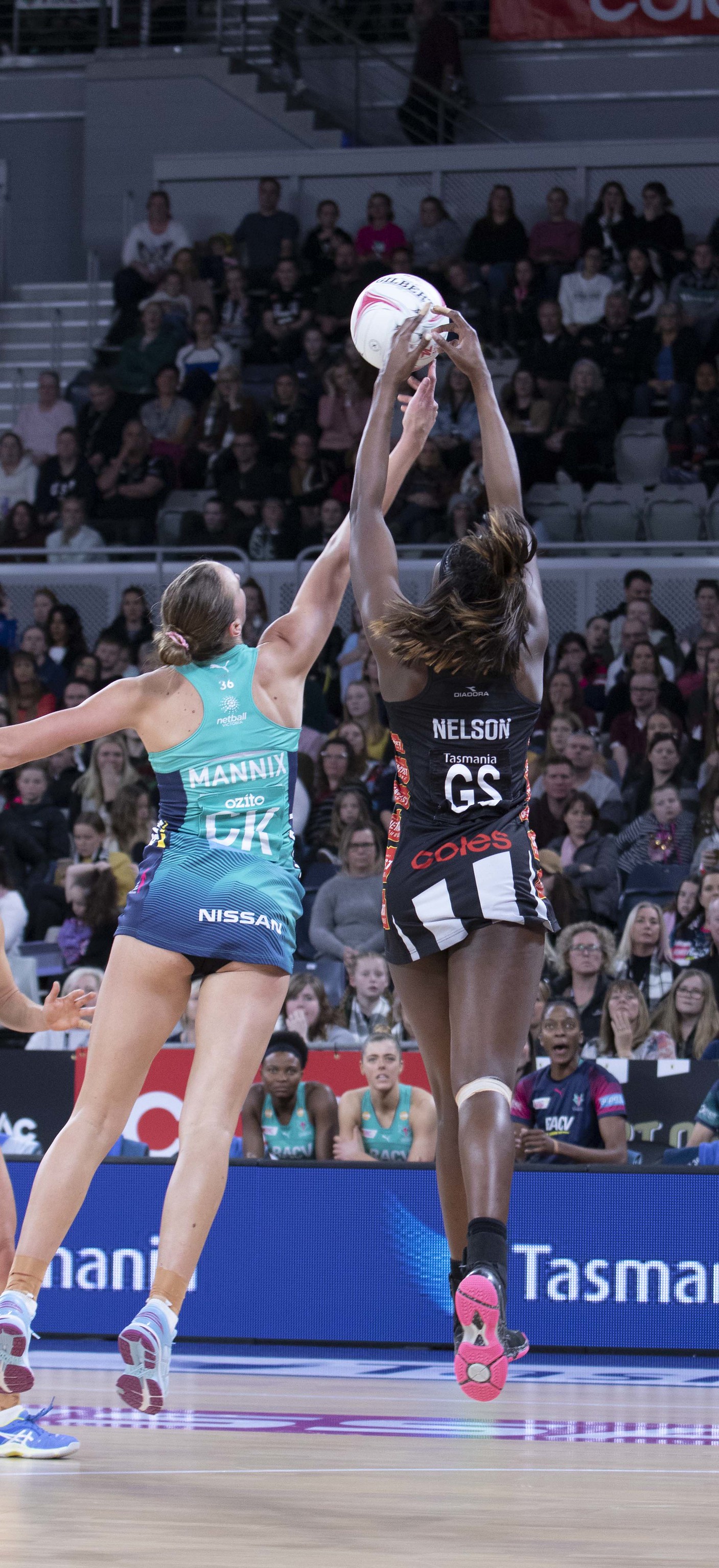In this dynamic photograph taken during an indoor volleyball tournament, two female players are caught mid-jump with their backs to the camera as they reach for a white volleyball. The player on the left, identified as Mannix, is wearing a blue tank top and very short black shorts, while the player on the right, named Nelson, sports a black jersey with matching shorts and shoes featuring pink soles. Both women stretch their right arms overhead towards the ball. The scene is set against a backdrop of two tiers of bleachers filled with spectators, who are partially in shadow. A blue barrier at the base of the bleachers displays the word "Tasmania" in white font, adding a splash of color to the wooden-floored court. The players are illuminated more brightly, drawing focus to their athletic form and the intense moment of the game.